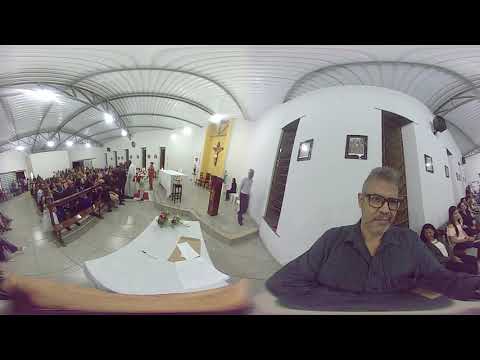This image is a 360-degree panoramic shot of an indoor church, captured through a Virtual Reality lens that causes some distortion, particularly noticeable in the vaulted ceiling with crisscrossing ribs or metal beams. The focal point is a raised dais situated against a central yellow wall, featuring a lectern on one side and what appears to be an altar with a crucifix on the other. Several individuals are present on the dais, including a man in blue pants and shirt stepping down. In the foreground, a man with gray hair, a beard, and glasses, dressed in a dark blue shirt, stands behind what seems to be a desk or a large altar. Around this desk are flowers and various items, though their connection to the dais and the altar setup is unclear. The congregation is relatively small, with people seated in pews and others with their backs against another wall. Additionally, a prominent figure on the right side of the image—a gray-haired man in a gray button-down shirt and black glasses—contributes to the scene, reflecting the communal aspect of this church service.